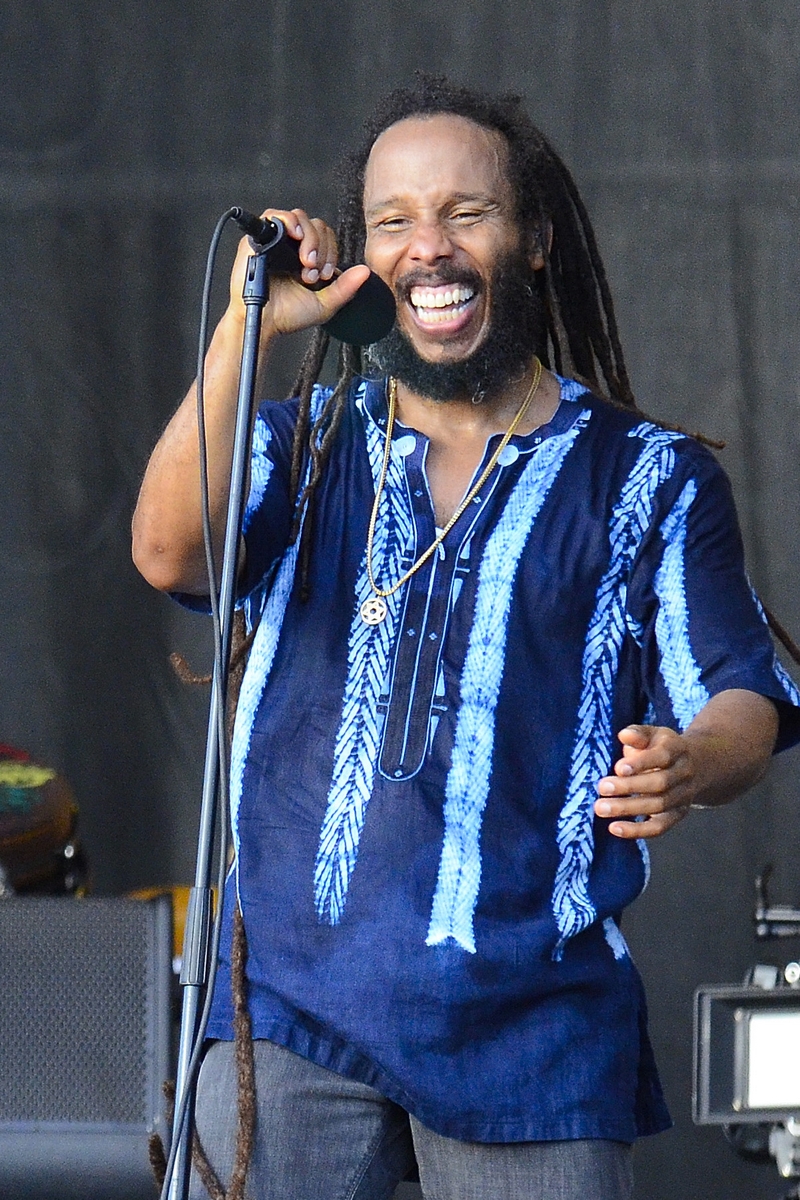The image captures a charismatic black performer with long dreadlocks and a thick black beard, smiling ecstatically as he holds a microphone in front of his face. The microphone is mounted on a stand. He is wearing a vibrant, tropical-looking blue button-up shirt adorned with intricate, white feathery or tie-dye-like stripes and patterns, paired with jeans. Around his neck, he sports a necklace. The scene unfolds on a stage, indicated by the presence of a speaker in the background and a gray brick wall. The performer is bathed in natural light, and the overall image is clear, highlighting the energy and focus of his performance.